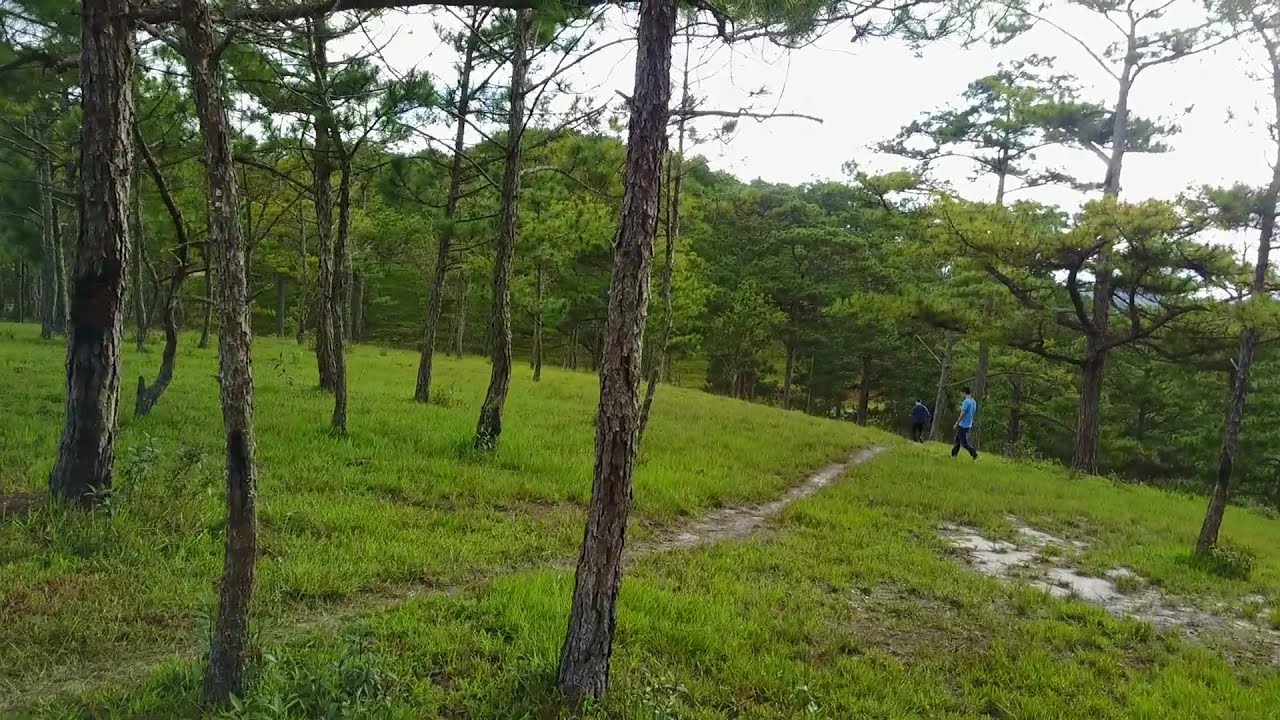In this serene forest park setting, the ground is covered with lush green grass and meandering through it is a very narrow, unpaved footpath that starts from the bottom left of the image, leading to the center and extending into the background. The grassland is dotted with many tall, thin trees whose peeling bark gives them a distinctive, textured appearance. These trees are sparsely spaced, with several feet between each one, and they have limited foliage, which makes the area look somewhat empty. In contrast, the trees in the far background are taller and denser, their full canopies creating a stark silhouette against the bright white sky. 

Amidst this natural scene, a man with dark hair is seen walking near the narrow path, wearing a light blue short-sleeved t-shirt and black pants, his hands resting at his sides, head down in contemplation. The foreground also hints at a history of human presence with an overgrown area on the bottom right, possibly the remnants of a small paved space or parking lot now reclaimed by nature, adding to the quiet and slightly overcast ambiance of the park.